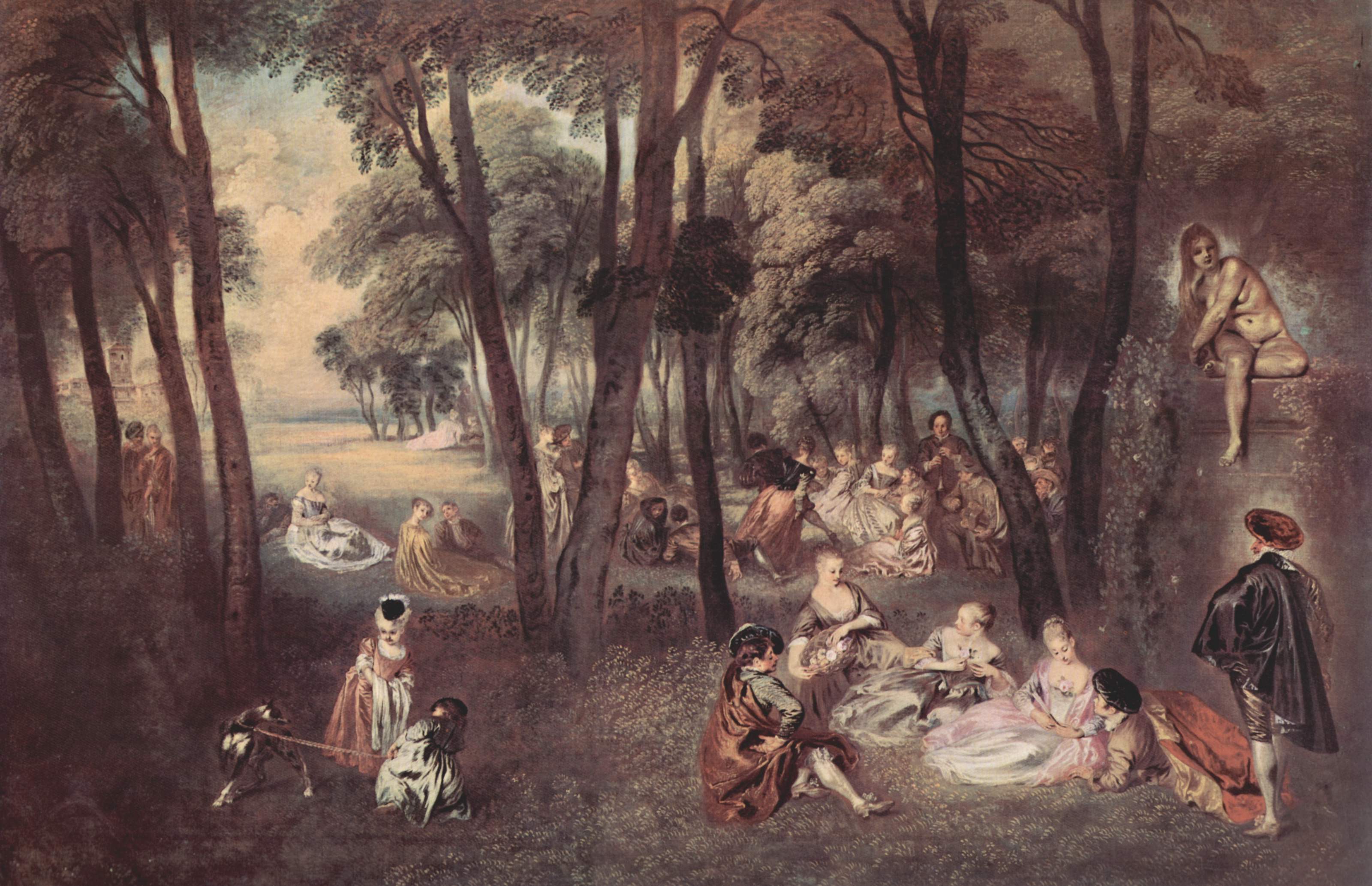The painting, "Entertainment Countryside" by Antoine Watteau, completed in 1718, is a captivating example of Rococo Pastoral style. It is a landscape-oriented, color oil painting that depicts a tranquil forest scene bathed in tones of browns, faded greens, and off-white hues. The scene illustrates various groups of people adorned in Victorian and Renaissance attire, gathered amidst the colorful trees and a park-like setting.

In the foreground to the left, two children are seen playing with a brown and white dog on a leash in a clearing. To the right, several women in full Renaissance dresses are seated on the grass, engaged in conversation, while two men look on. A standing man with a black cape over his shoulder gazes into the distance, his back turned to a voluptuous, nude, blond-haired woman with her arm laid across her and one leg underneath the other. She is perched on a concrete platform entwined with ivy, overseeing the scene from above.

In the background, groups of people sit and converse in a semicircle, enhancing the painting's communal atmosphere. Amidst the right edge, an ethereal, angelic figure appears to levitate, adding a touch of mysticism to the serene tableau. The painting's detailed composition and harmonious hues reflect the playful elegance characteristic of Watteau's Rococo influence.